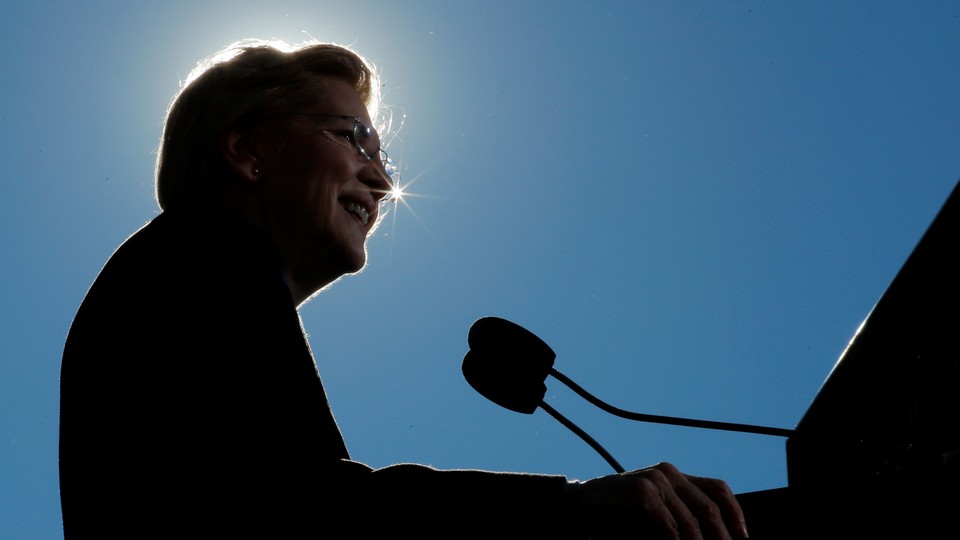This photograph captures Senator Elizabeth Warren in a striking, high-contrast silhouette as she stands at a podium, giving a speech under a clear blue sky. The image is taken from a lower angle, looking up, which positions her directly in front of the sun, creating a radiant halo effect around her head and casting her features mostly in shadow. Her short, combed-back hair, circular earrings, and glasses, which feature prominent lens flares, are visible. Despite the heavy shadow, her smile is discernible as she faces what appears to be an audience. Warren's hands grasp the sides of the podium, and two microphones with black coverings are pointed towards her. The intense sunlight creates a stark white light surrounding her head, making the photo especially stylistic and high-quality. Her dark sport coat blends into the shadow, leaving just the details of her hands and faint hints of her expression illuminated.